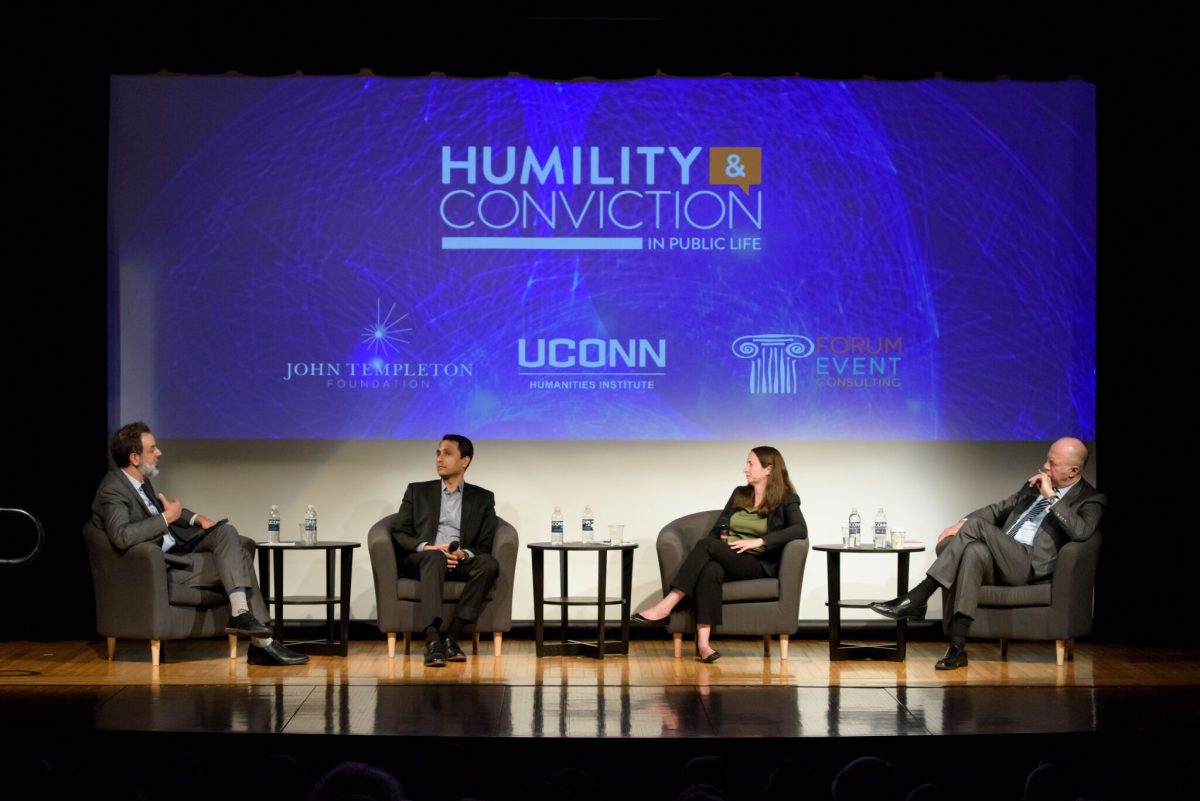This is a detailed color photograph in landscape orientation capturing a live panel discussion on a wooden stage, situated within an indoor convention hall. The stage features four individuals seated in chairs—three men and one woman—from left to right. The first man on the far left, dressed in a gray suit with a shirt and tie, has a gray beard and dark hair and is currently speaking to the second man. This second man, who has dark skin and dark hair and is wearing a black blazer with a gray shirt and black pants, holds a microphone in his hand but is listening attentively. The third person is a woman with long brown hair, dressed in a black suit with a green shirt, who also has her legs crossed and is looking towards the two men engaged in conversation. The fourth individual, a man with a receding hairline in a gray suit, white shirt, and tie, is also sitting with his legs crossed, attentively listening. Between each pair of chairs are tables holding two bottles of water each.

The background features a large blue screen displaying the words "Humility and Conviction in Public Life" along with logos for John Templeton, UConn, and another event center, indicating this is a formal presentation or discussion organized by these entities. The overall photographic style is representational realism, emphasizing the professional and structured setting of the event.